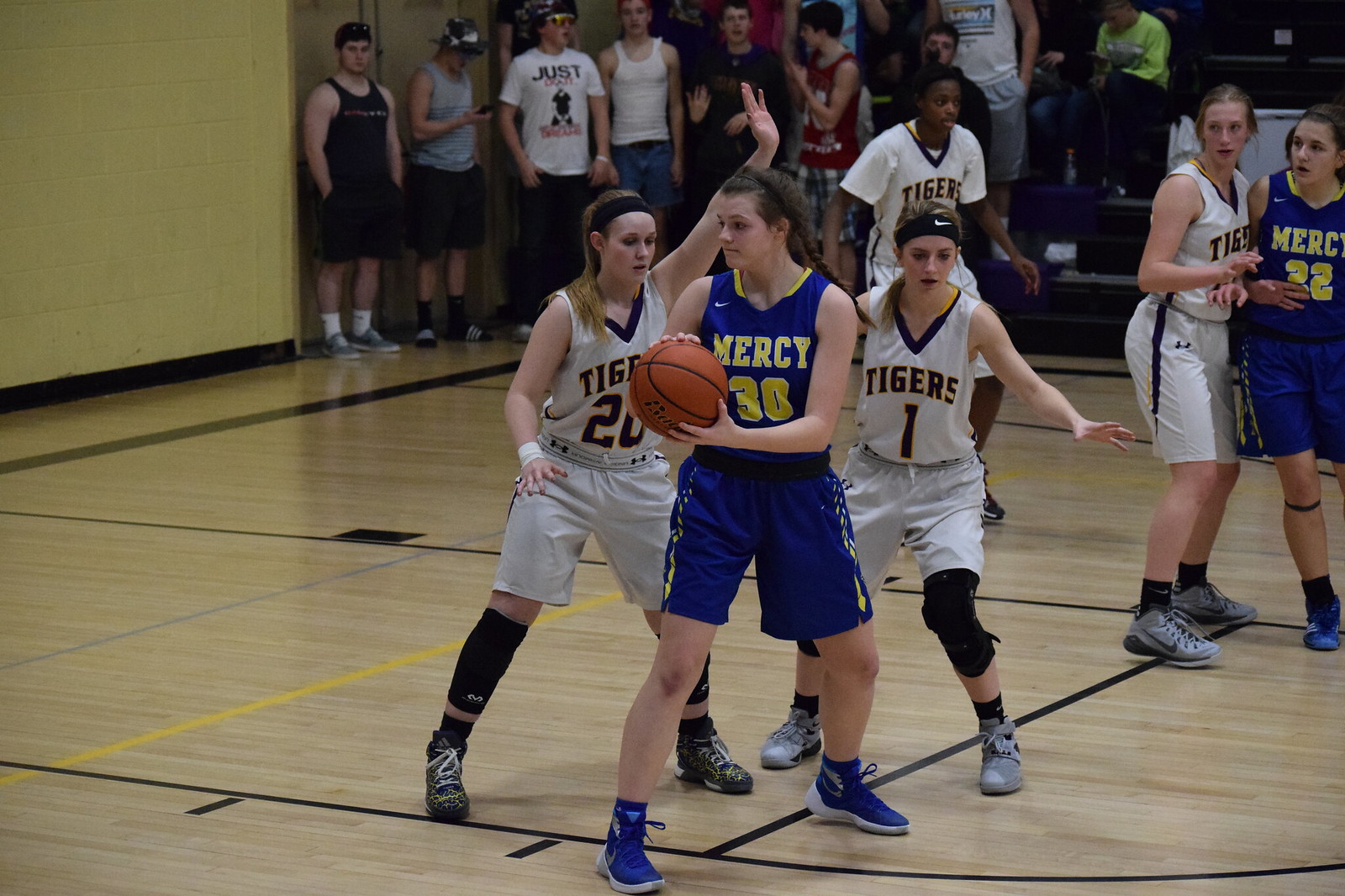Inside a brightly lit gymnasium with yellow-painted walls and tan wooden floors, an intense girls' basketball game unfolds. The team in blue uniforms with yellow lettering, known as Mercy, faces off against the Tigers, clad in white uniforms with black lettering. In the foreground, Mercy's number 30, dressed in blue with matching shoes, holds the basketball at waist height. She faces the viewer, but her head turns to the right, focused on the play. Directly in front of her, Tigers' number 20 defends, with her left arm raised and her right arm, adorned with a white wristband, positioned at waist level. To the left shoulder of number 30, another Tigers player, number one, sporting a black Nike headband and a ponytail, stands with her arms extended and wearing black knee pads. To the right of this trio, additional players from both teams are visible – one in blue and one in white. In the background, around 10 to 12 teenage boys dressed casually in shorts, pants, and t-shirts stand near the bleachers, some wearing hats and one donning glasses, intently watching the action on the court.